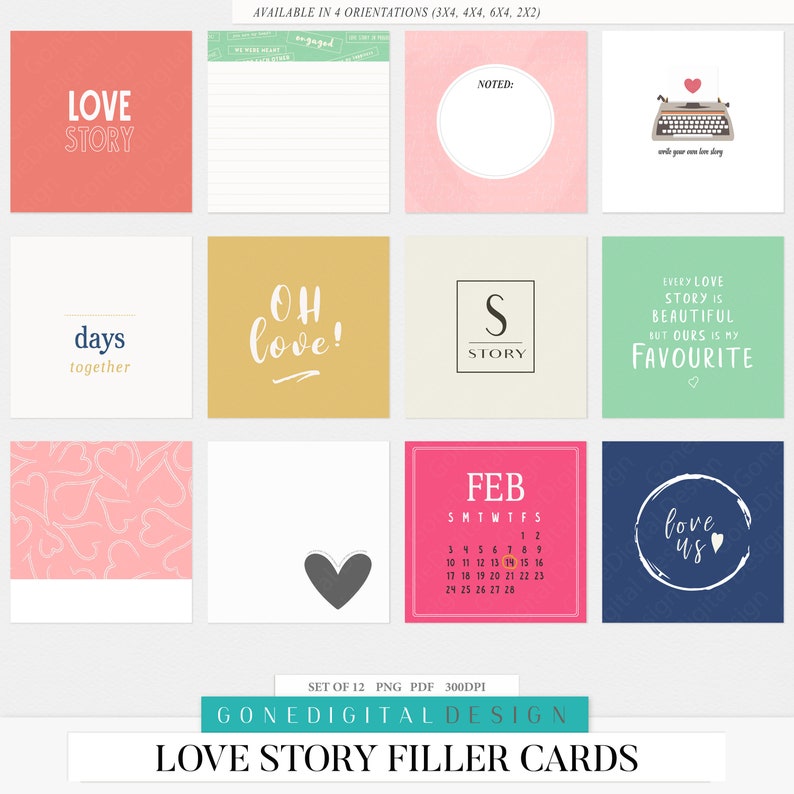The image is a photograph of an advertisement set against a grayish background. At the top right corner, there's a small bar featuring text that reads, "Available in four orientations" followed by the dimensions: 3x3, 3x4, 4x4, 6x4, and 2x2. The main section of the advertisement showcases twelve card designs arranged in three rows of four cards each. These cards are slightly taller than they are wide.

In the first row from left to right:
1. A red card with the phrase "Love Story" in white text.
2. A white card that resembles lined paper with a green strip at the top.
3. A pink card with a white circle in the middle featuring the word "No" at the top.
4. A white card depicting a typewriter with an envelope and a red heart coming out of it.

In the second row from left to right:
1. A white card with the text "Days Together."
2. A golden card with the exclamation "Oh, Love!"
3. A white card with a black box containing the words "S Story."
4. A green card with the text "Every Love Story is Beautiful, But Ours is My Favorite."

In the third row from left to right:
1. A card that is partially pink with heart designs and a white strip at the bottom.
2. A white card with a black heart situated at the bottom right-hand corner.
3. A pink card displaying the word "February" above a calendar layout.
4. A dark blue card with a circle containing the words "Love Us" and a heart symbol inside.

Overall, the advertisement is a colorful assortment of creative and romantic designs, each card presenting a unique message or illustration.